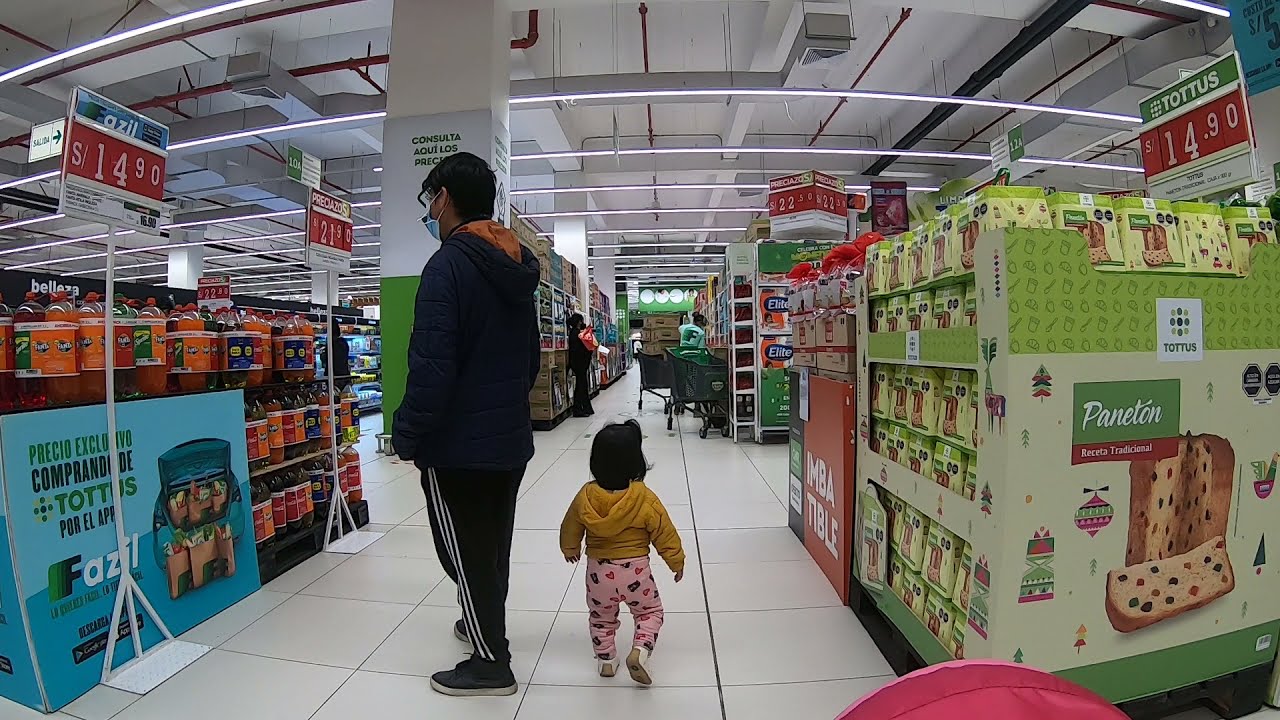The image captures the interior of a large warehouse-type grocery store, well-lit with fluorescent ceiling lights and featuring wide, white linoleum tile flooring. Centrally positioned is a man of Asian descent wearing a dark blue or black puffy jacket with an orange-lined hood. He has dark hair and wears a blue turquoise mask. His outfit is completed with black track pants featuring white stripes running down the sides and black trainers with white soles. Standing next to him is a young child, likely around three years old, dressed in a gold-yellow jacket, pink pajama bottoms with heart prints, and white shoes.

To the left of the scene, there is a display of large two-liter soda bottles in orange and red hues. On the right side, a boxed structure with shelves is filled with Panettone, traditional Italian bread, marked with a red sign bearing the price $14.90. Nearby, several more grocery aisles stretch into the distance, populated by a few other shoppers. Notably, one shopper in a green jacket and another in all black are pushing shopping carts stacked with various items. In the background, another person, partially obscured, is visible at the far end of an aisle. The store signage includes multiple red and white price tags, such as $21.00 and $2.19, enhancing the detailed and active atmosphere of this bustling grocery store.